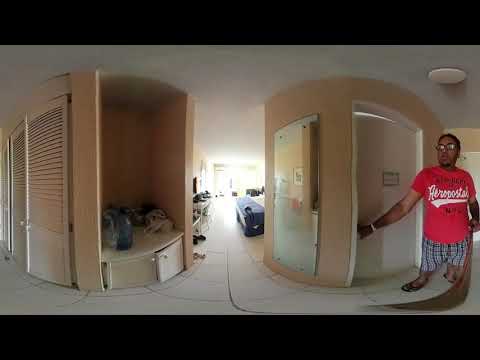This panoramic 360-degree photograph showcases the interior of a home with soft tan-colored walls and white square-tiled flooring accented with dark grout. Central to the image is a hallway leading to a larger room, partially obscured by bright sunlight streaming in through windows. On the far right, an Indian-looking man with darker skin, wearing glasses, a red T-shirt with white letters spelling "AEROPOSSILE," plaid shorts, and flip-flops, is seen opening a white door. He appears to be looking straight ahead but slightly to the left. The hallway features more wood doors on the left, and an alcove cluttered with random items. A small closet with a shelf at the bottom can also be noticed along the left wall. The space is filled with round, circular wall formations, contributing to the panoramic warping of the image.